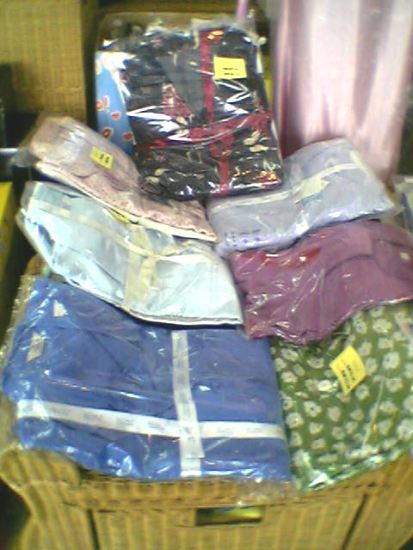This slightly out-of-focus photograph captures an indoor setting featuring a yellow-walled room with a shiny pink curtain hanging on the right. Central to the scene is an overhead view of a wicker basket, which includes a visible drawer at the bottom. The basket, in a yellowish-brown tone, is filled with various garments or sheets, all individually packaged in clear plastic protectors that may still be in their original packaging, as evidenced by the yellow stickers on some of them, though the text on the stickers is not discernible. The garments come in a myriad of colors: there's a lavender-colored piece, a maroon one, a green garment with white floral patterns, a pink, a light blue, and a blue one adorned with white ribbons. A black fabric with red and gold floral patterns can be seen towards the back, and another description notes a blue garment with white bands, potentially hinting at designs that blend into each other. Together, these elements create a vibrant and textured display, suggesting the contents might be for sale in what seems to be a retail environment.